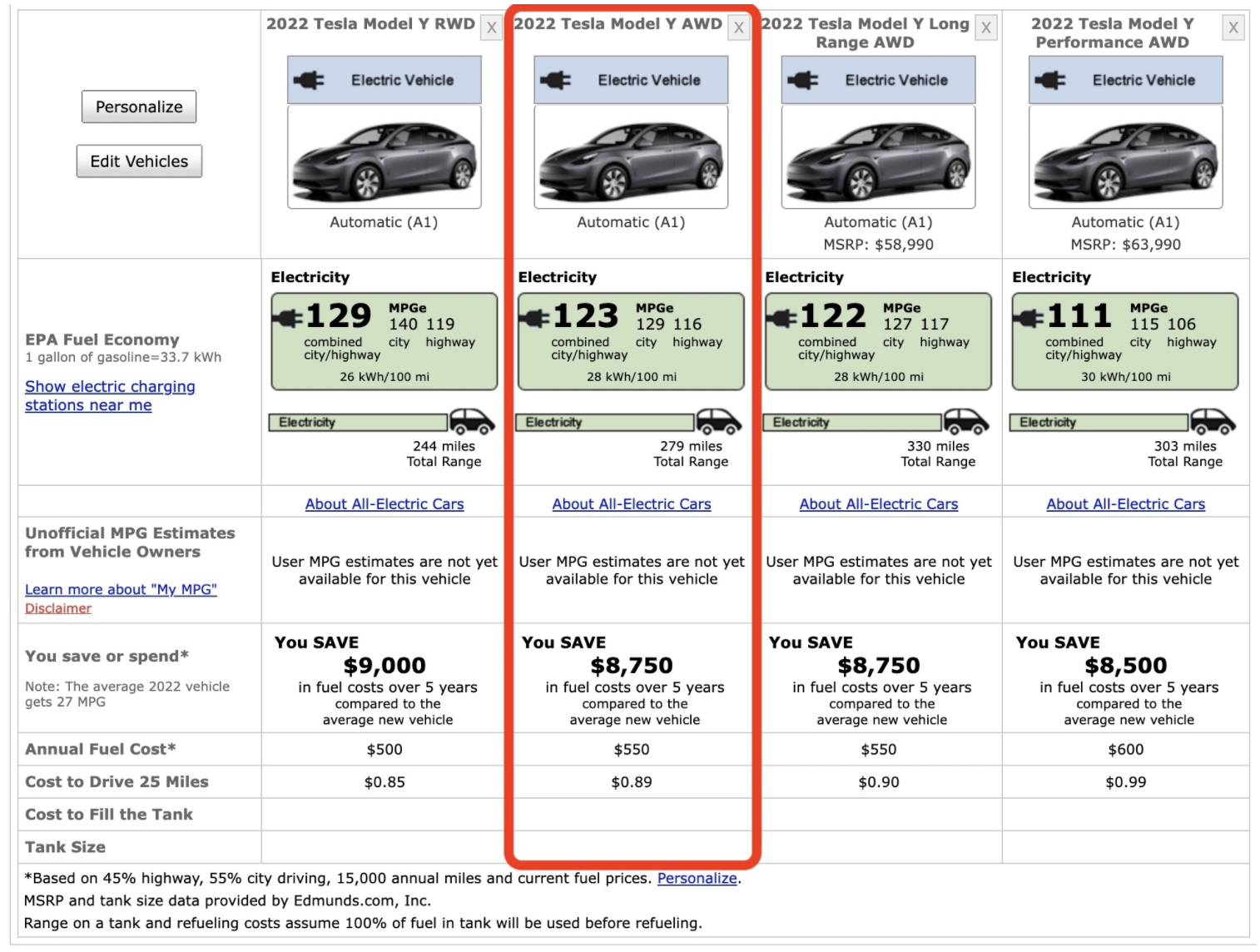The image features a webpage, possibly resembling a layout similar to Craigslist, where four Tesla Model Y vehicles are displayed. At the bottom of the page, there is a note stating: "MSRP and text size data provided by Edmunds," indicating that the information may have been sourced from Edmunds. 

The showcased vehicles include a variety of Tesla Model Y versions, identified as either rear-wheel drive or all-wheel drive, with specific models highlighted as 'Long Range' and 'Performance.' All the Teslas appear in silver and are fully electric, boasting impressive electric vehicle (EV) mileage figures. The best mileage listed is 129 MPG equivalent (MPGe), with the lowest being 111 MPGe.

Additionally, a section on the page discusses potential savings, indicating that owners could save between $8,000 to $9,000 in fuel costs over five years when compared to the average new vehicle. However, the actual prices of the cars are not visible in the image.